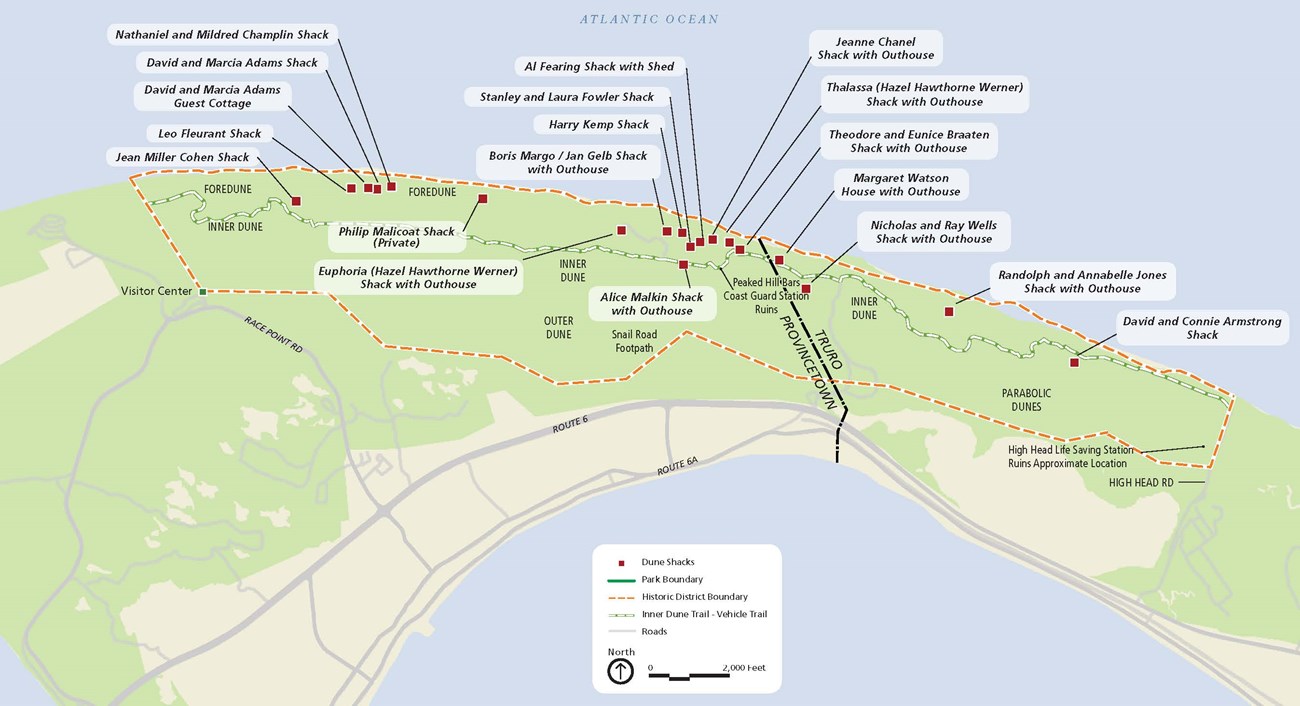This detailed map depicts Provincetown, a location surrounded by the light blue expanse of the Atlantic Ocean. The map prominently features Route 6 and has numerous named sites primarily concentrated along the coastline and within dune areas. Among the notable locations are Dave and Connie Armstrong Shack, Randolph and Annabelle Jones Shack without house, Theodore and Eunice Bratton Shack without house, Al Fearing Shack with shed, Philip Malakote Shack private, Hazel Hawthorne Werner Shack with outhouse, and the Visitor Center. The map also identifies geographical features like Inner and Outer Dunes and Parabolic Dunes, as well as Peaked Hill and Peaked Hill Bars Coast Guard Station Ruins.

The cartographic details include symbols and colored lines: dune shacks marked with red squares, the park boundary delineated by a green line, and the historic district boundary shown with yellow dashes. The roads are clearly marked, including Rage Point Road, and trails are indicated for both inner dune and vehicle access. A legend is included for context, specifying scale (2,000 feet), and an arrow points north. The map is shaded with light blue for the ocean, gray for park areas, and pinkish hues delineate certain regions, interconnected by blue roads. Additionally, it names Truro and Provincetown, situating the map's precise location.